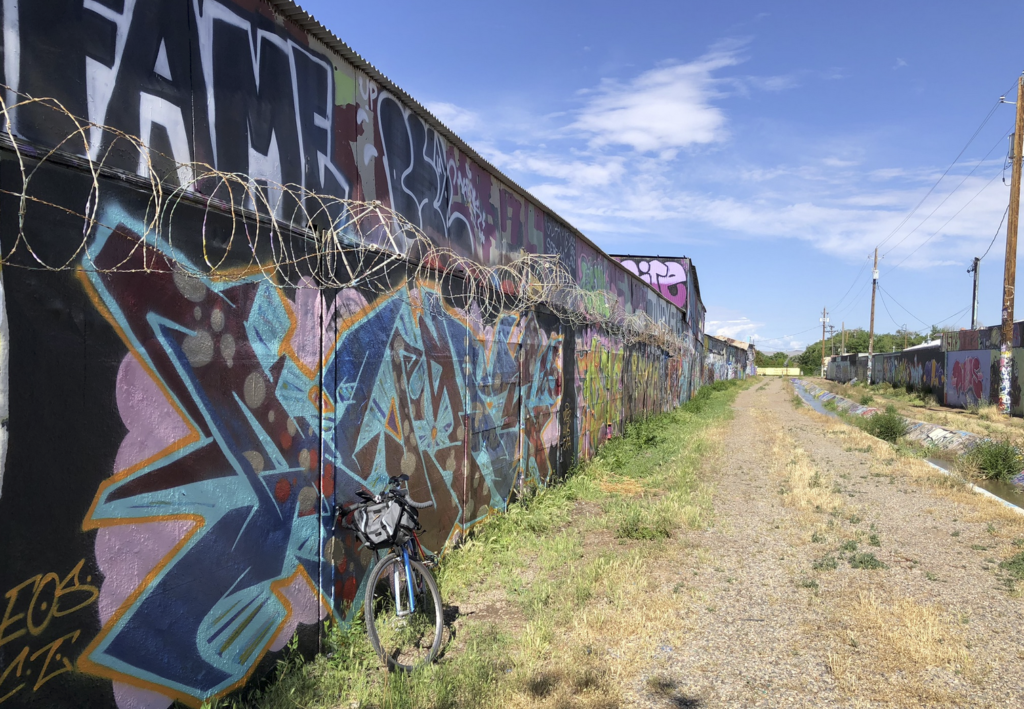The photograph captures a seemingly abandoned area dominated by a tall, two-tiered wall covered in vibrant graffiti. The wall, potentially built up over time, is adorned top to bottom with layers of tags, primarily featuring the work of an artist identified as "EOSCJ" and the word "FAME" prominently displayed at the top. A blue 10-speed bicycle with a travel bag attached to its handlebars rests against this graffitied wall. About two-thirds up, a rusty row of spiral barbed wire stretches off into the distance. 

In front of the wall, a gravel road, interspersed with overgrown weeds and brush, parallels a cement irrigation ditch that appears to contain some water and has plants lining its edges. On the opposite side of this ditch are power poles extending into the distance, also decorated with graffiti. Beyond these poles, another patchwork-like wall is visible, adding complexity to the scene with its own set of colorful tags. 

The sunny sky, with a few scattered clouds, illuminates the area, casting light on the trees in the background, indicating a bright and open environment. The combined elements of graffiti, the bicycle, and the surrounding structures create a rich narrative of urban decay and artistic expression.